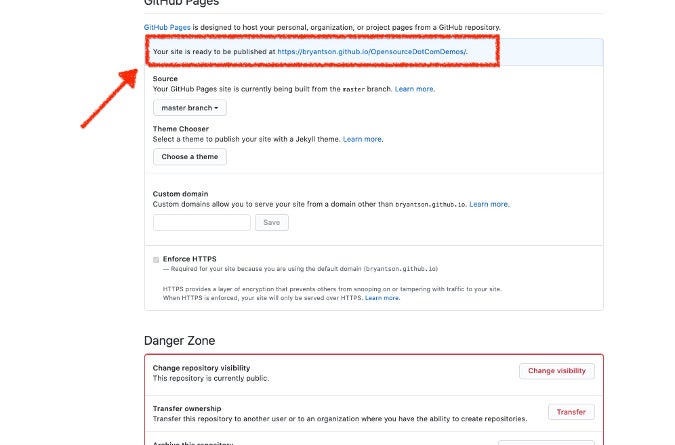### Detailed Caption for the Image:

The image is a screenshot of a GitHub information page specifically for GitHub Pages settings. At the top left corner, the partially visible title reads "GitHub Pages." Below the title, a description states: "GitHub Pages is designed to host your personal, organization, or project pages from a GitHub repository."

A prominent feature in the middle of the page is a red rectangular box containing the message: "Your site is ready to be published at" followed by a link to "bryantson.github.so." To the left of this red box, a red arrow highlights the message indicating the site's readiness.

Beneath the red box, there is a section labeled "Source." This section specifies that the GitHub Pages site is currently being built from the "master" branch of the repository. The master branch is selected as the source, displayed clearly within this section.

Further down, there's a "Theme chooser" section, which allows the user to select a Jekyll theme for the site. At the moment, no theme has been chosen.

Continuing down, there's an option for "Custom domain," though no domain has been entered in this field.

At the very bottom of the page, there is a "Danger Zone" section, outlined in red. This section includes options such as "Change repository visibility" and "Transfer ownership," presumably for emergency scenarios or significant administrative changes to the repository.

The entire layout visually guides the user through the necessary settings to configure and publish their GitHub Pages site, with key areas emphasized using red boxes and arrows.